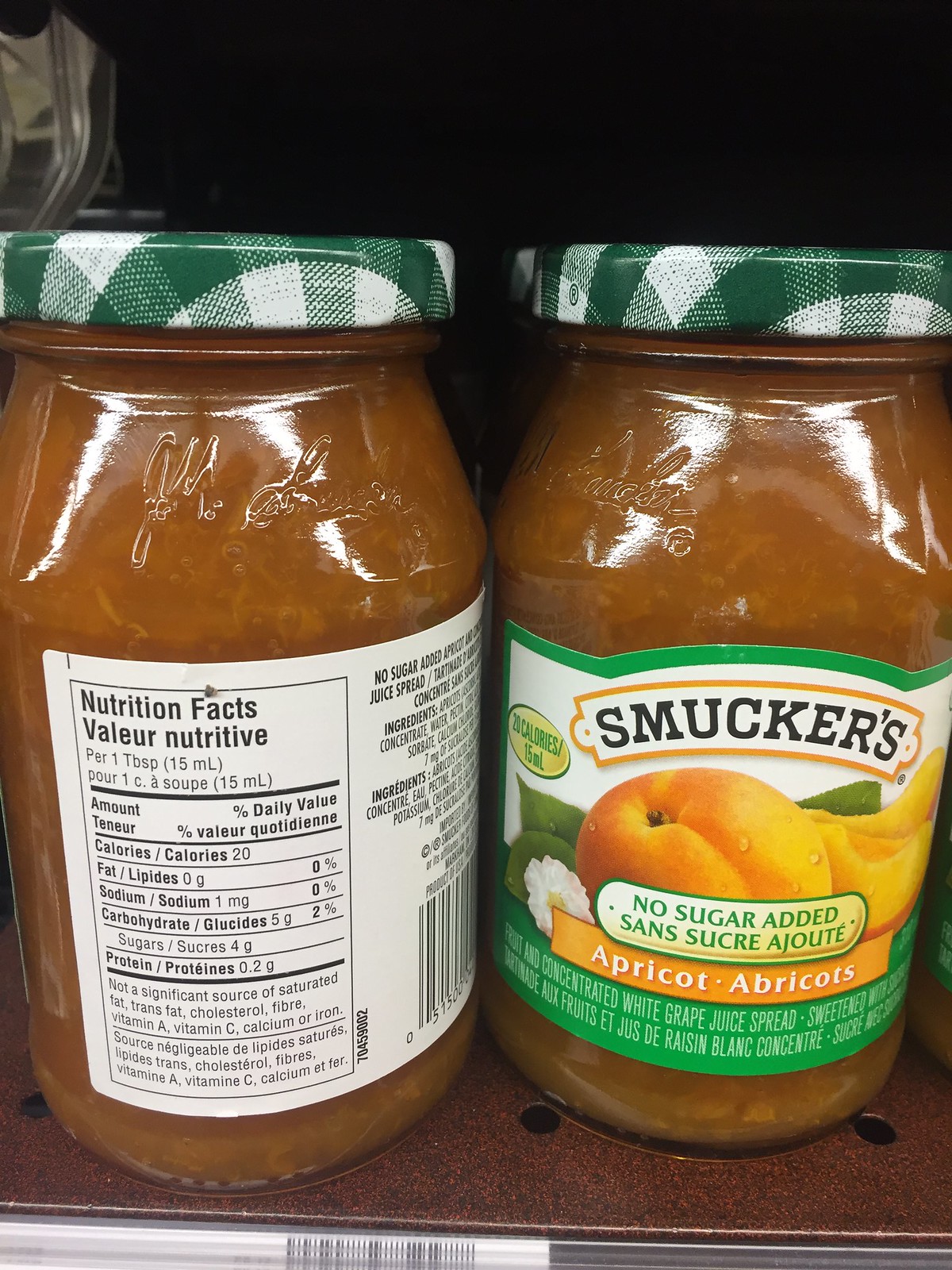This detailed photograph captures two clear glass jars of Smucker's No Sugar Added Apricot Preserve, prominently displayed on a dark brown supermarket shelf amidst rows of similar jars. The main focus is on the jar to the right, showcasing the front label that reads "Smucker's" in black text, accompanied by an illustration of apricots and the inscription "No sugar added sans sucre ajouté." The jar on the left is rotated to reveal the nutritional facts on a white label, indicating information per one tablespoon such as calories, fat, sodium, carbohydrates, sugars, and protein. The preserves inside the jars appear thick and brown, with visible chunks of apricot. A barcode on a white tag is visible at the bottom of the shelf, adding to the retail context of the image.